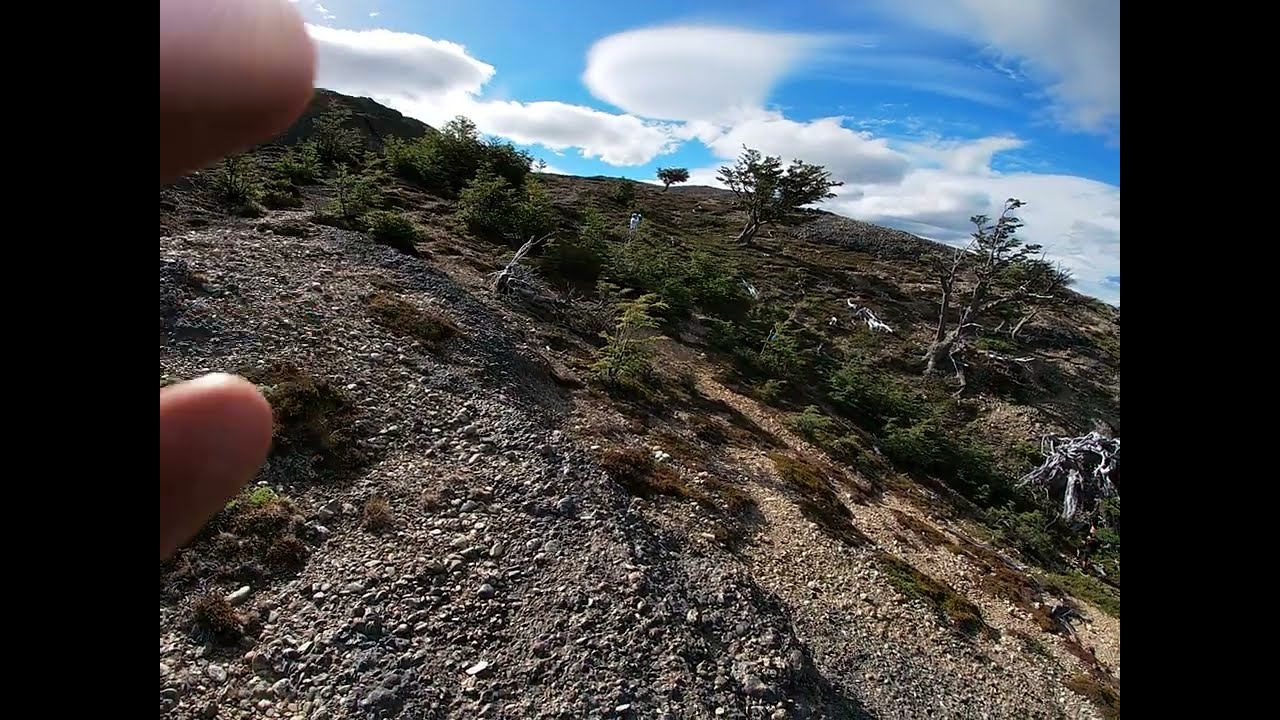The photograph captures an imposing hillside from a low perspective, looking upward toward a bright blue sky infused with scattered white clouds. The foreground showcases a mix of light and dark gray gravel interspersed with patches of green and brown moss. To the left and center, scattered bushes and vibrant green shrubbery accent the rocky terrain, while the right side is dominated by stumpy trees and grass. Part of the photographer's fingers obscure the top-left and center-left sections of the image, suggesting an inadvertent inclusion while holding the smartphone. Black ribbons along the left and right edges, likely artifacts from a website or cropping, frame the scene, which is devoid of any identifying landmarks or trails. The sky above the hillside suggests daytime with potential wind activity, as evidenced by the form of the clouds. Overall, the image displays a raw and untouched chunk of nature, juxtaposed with the minor human element of the fingers.